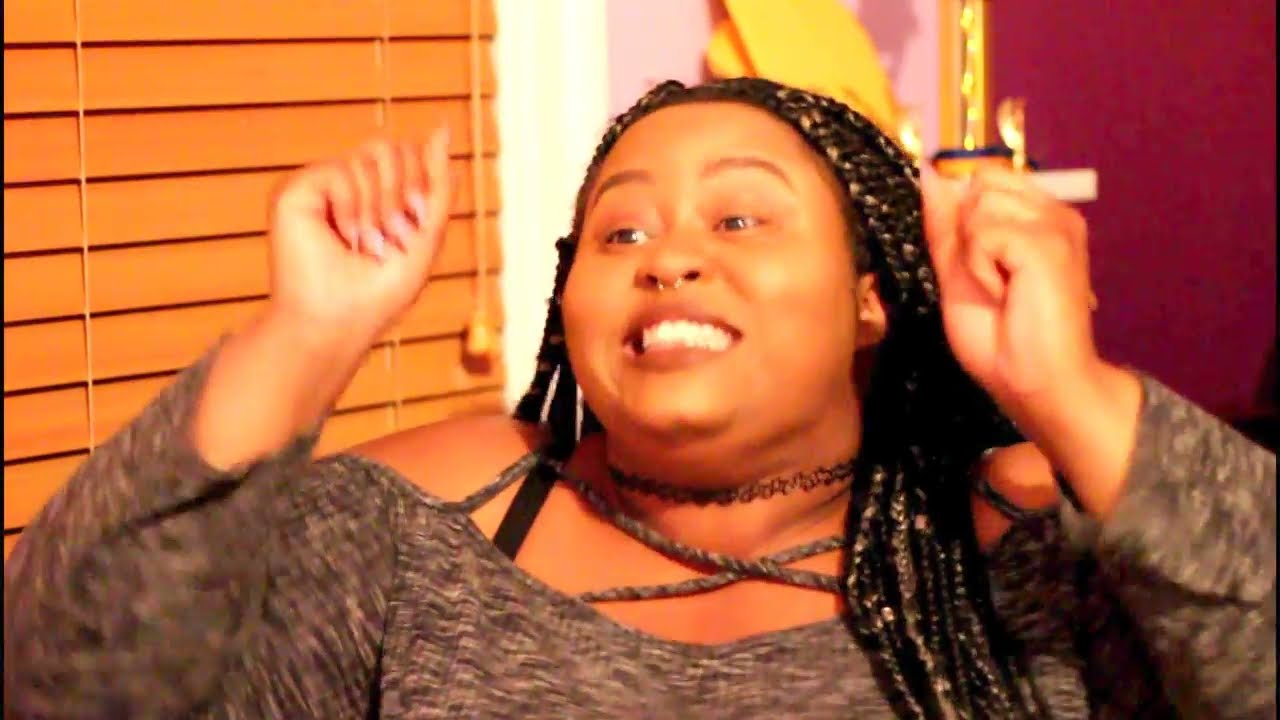In this image, a heavyset Black woman is positioned centrally, exuding palpable excitement. Her face is the focal point, directly in the center of the frame, with her eyes narrowed in joy and eyebrows raised. She's smiling broadly, displaying her teeth, and has her hands raised near her face, with closed fists that convey happiness rather than anger. She is adorned in a gray, off-the-shoulder sweater that drapes comfortably, and her long black hair is elegantly braided with finery, cascading over her right shoulder.

The backdrop features a blend of interesting details: to the left, light brown wooden blinds are visible, slightly slanted and closed. Directly behind her head, the wall is adorned with a vibrant artwork characterized by hues of gold and pink. Adjacent to this artwork on the upper right side of the image, the wall continues in a deep, rich maroon color, creating a visually appealing contrast. The scene is set indoors, likely in a living room, capturing a moment of pure, jubilant excitement. The predominant colors in the image are orange, gray, brown, black, yellow, gold, and maroon, adding warmth and richness to the setting.